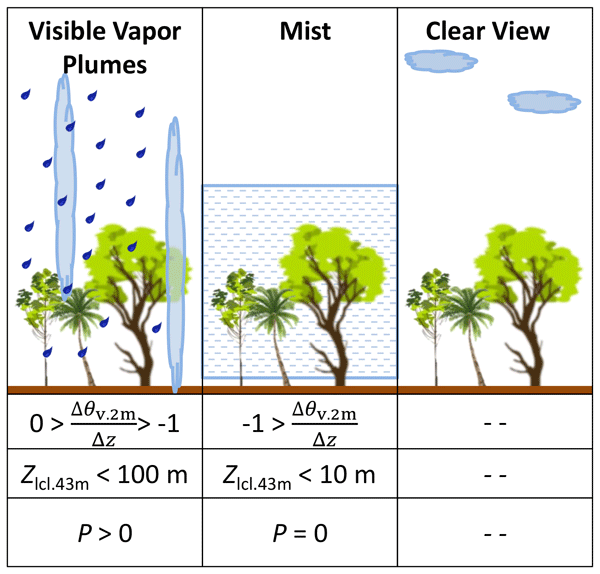The image is a detailed scientific diagram split into three vertical sections with a white background and thin black borders. Each section represents different atmospheric conditions affecting three green trees growing from a brown soil line. 

On the left, the section titled "Visible Vapor Plumes" features blue raindrop-like dots and vertically oriented elongated ovals resembling vapor plumes falling from the sky. Below this visual, a mathematical equation is present stating "0 > ΔθV 2m / ΔZ > -1," followed by another box indicating "Z," with accompanying subtext "LCL 0.43m < 100m," and "P > 0."

The middle section labeled "Mist" depicts the trees enveloped in a misty rain, represented by thin horizontal blue dashes. This section also includes equations at the bottom, concluding with "P = 0."

The right section, titled "Clear View," shows two blue clouds positioned above the trees with no precipitation. Below this are simple dash marks instead of equations, emphasizing an unobstructed atmospheric condition.